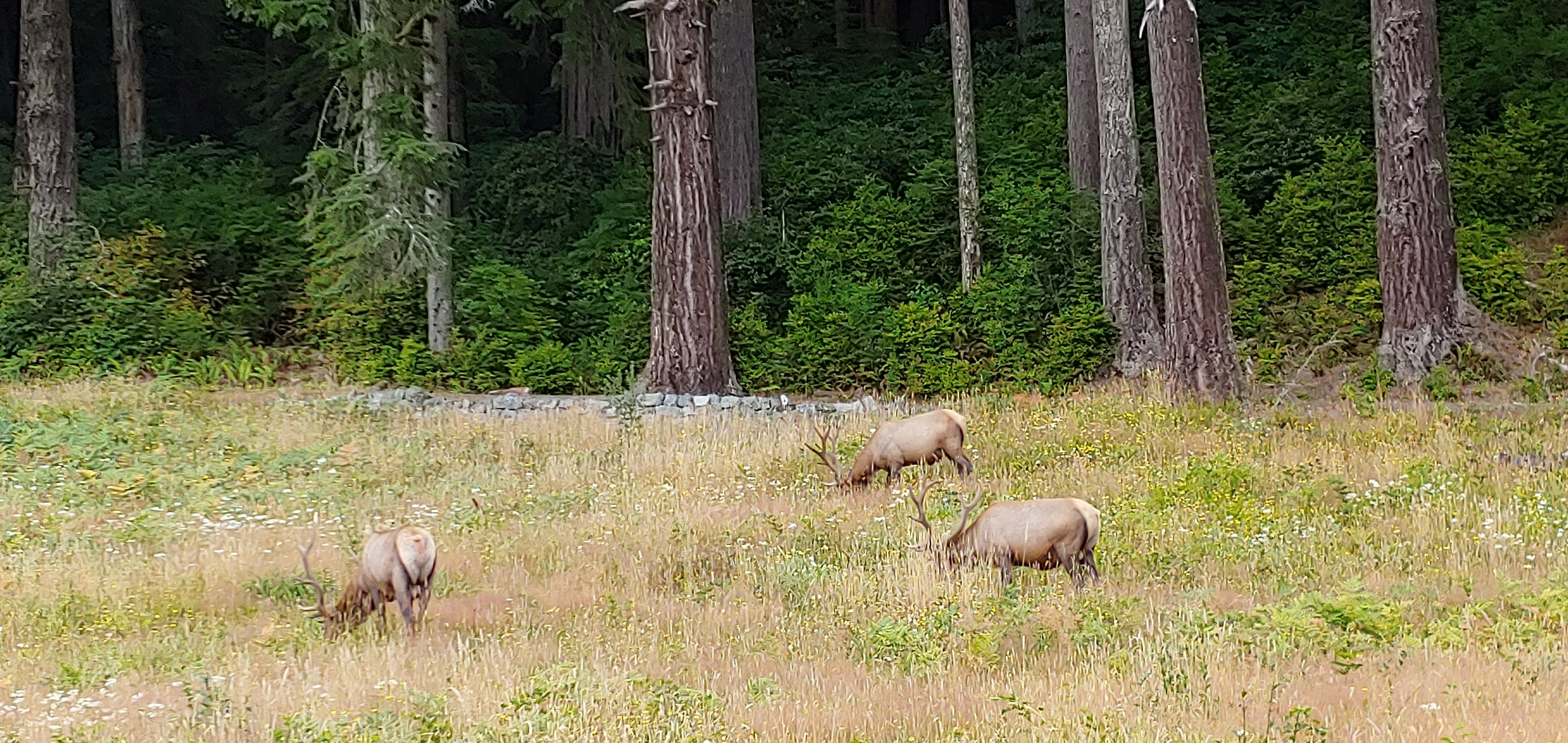In this detailed wildlife nature photograph, three fully-grown adult male elk are depicted grazing amidst a field of tall grasses and white flowers. The elk, distinguishable by their long, light brown antlers, dark brown hide, and comparatively lighter brown hind fur, are arranged with two feeding in the center and one off to the left. The grasses in the field vary in color, with some blades appearing dried and straw-like, while others are lush and green. The scene is set against a lightly lit daytime backdrop, with the sunshine possibly diffused by clouds, lending a gentle illumination to the setting.

Behind the elk, a stone wall partially demarcates the boundary between the field and a densely wooded forest. The forest is composed of a variety of tall trees with thick trunks spaced around 20 feet apart, and shorter green bush plants adding density to the forest floor. These tall trees provide a vivid green border, contrasting sharply with the dried grasses and indicating the untamed wilderness beyond. The elk, with their heads down and antlers rising from the grass, create a perfect focal point against this richly detailed, serene natural landscape. This offers a vivid portrayal of these majestic creatures in their natural habitat, poised on the edge of a dense forest where they can quickly blend into the thick greenery.